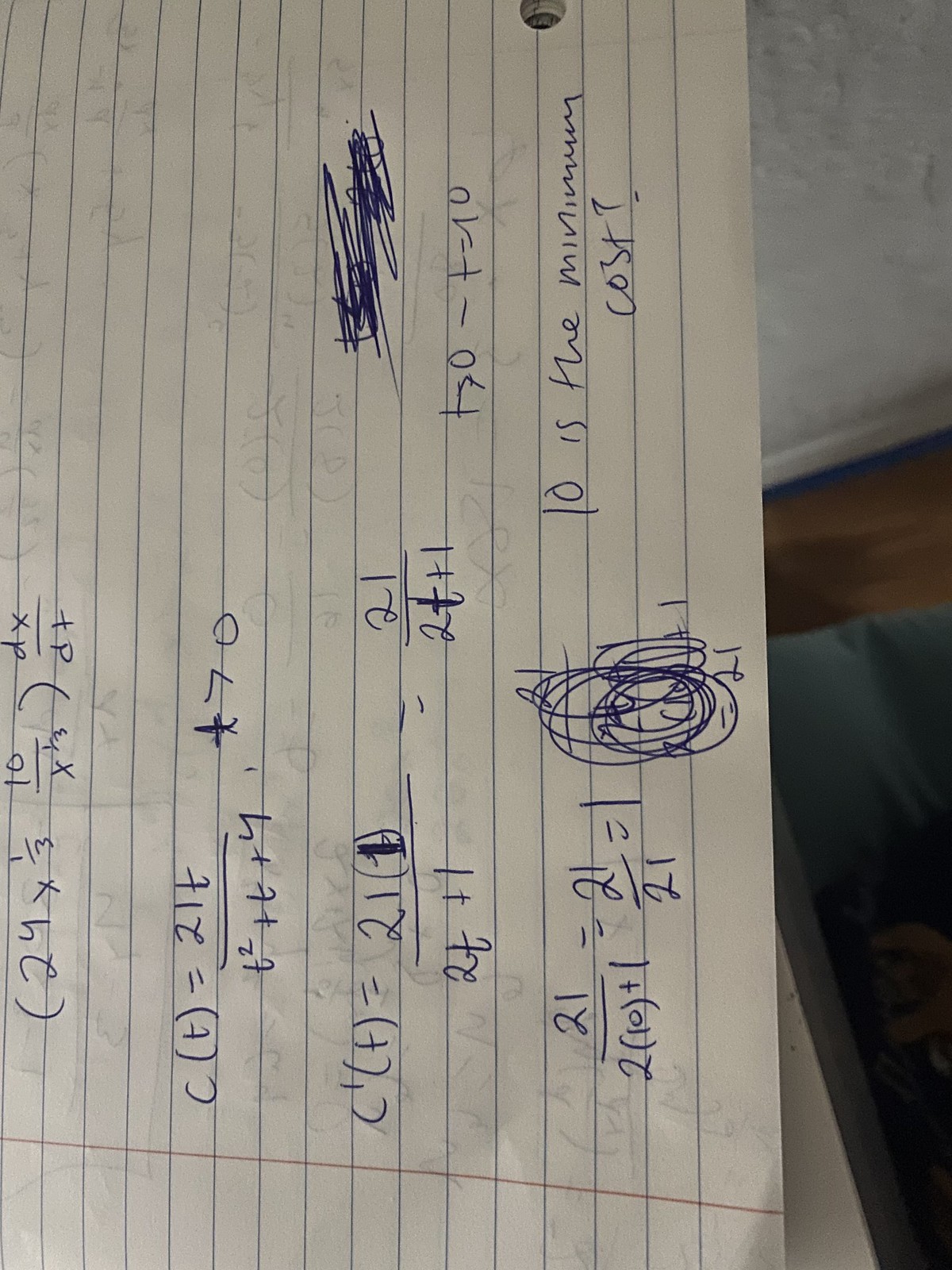The image captures a detailed segment of a college-ruled notebook paper featuring math homework. The paper is oriented sideways, displaying a portion of what appears to be the lower half of the page, or possibly the upper half flipped upside down. The visible part of the page is filled with handwritten math problems, penned in blue ink, and marred by several scribbles where errors were corrected. Notable equations include "24 × 1/3," "C(T) = 21T / (T² + T + 4)," and a step-by-step simplification of "21 / (2 × 10 + 1) = 21 / 21 = 1." Towards the opposite side of the paper, the phrase "10 as the minimum cost?" is clearly inscribed, indicating the student's query about a cost calculation problem.

Behind the paper, glimpses of the immediate surroundings are visible. The right edge of the frame reveals part of a dark gray or blue floor and a brown wooden chair with a light gray cushion. The faint impressions of more mathematical work are visible through the paper, hinting at a continuation of similar calculations on the unseen side. The overall composition suggests a snapshot of a diligent student's math homework session.

This detailed scene captures not only the academic focus but also the setting in which the learning occurs, providing a glimpse into the student's workspace.